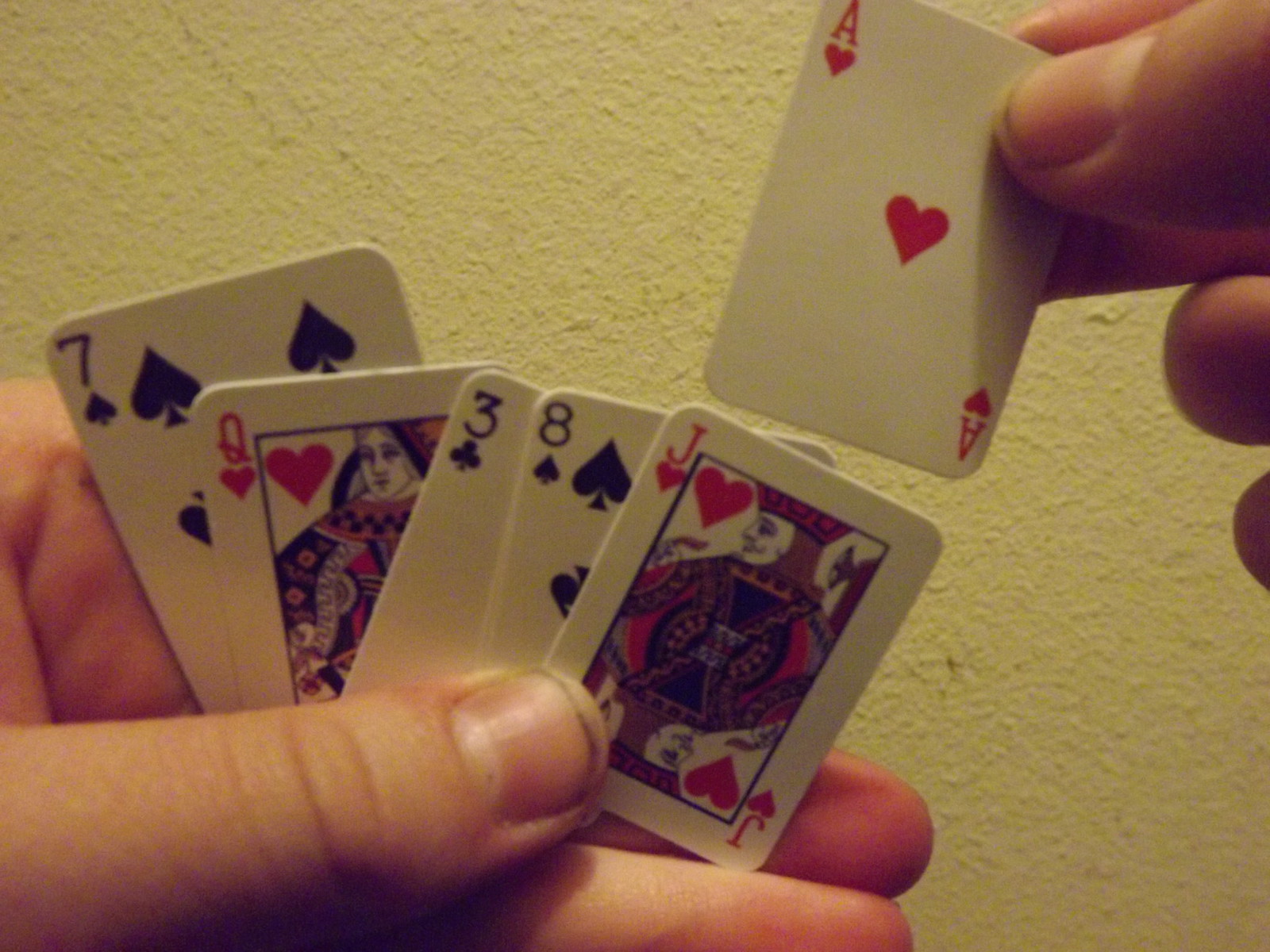In this image, an individual is holding a fanned-out hand of miniature playing cards against a pale yellow wall illuminated with a warm light. The person's left hand is prominently featured with their thumb in the foreground, showing a nail that appears to need cleaning. The hand displays six cards: the Seven of Spades, Queen of Hearts, Three of Clubs, Eight of Spades, Jack of Hearts, and the Ace of Hearts, which is held separately in their right hand. Both the left and right thumbs have noticeably dirty nails. The cards appear to be from a mini deck, indicated by their small size, and are slightly messily fanned, with the Seven of Spades on the far left and at the back of the fan. The Ace of Hearts seems to be in the process of being played or returned to the deck.